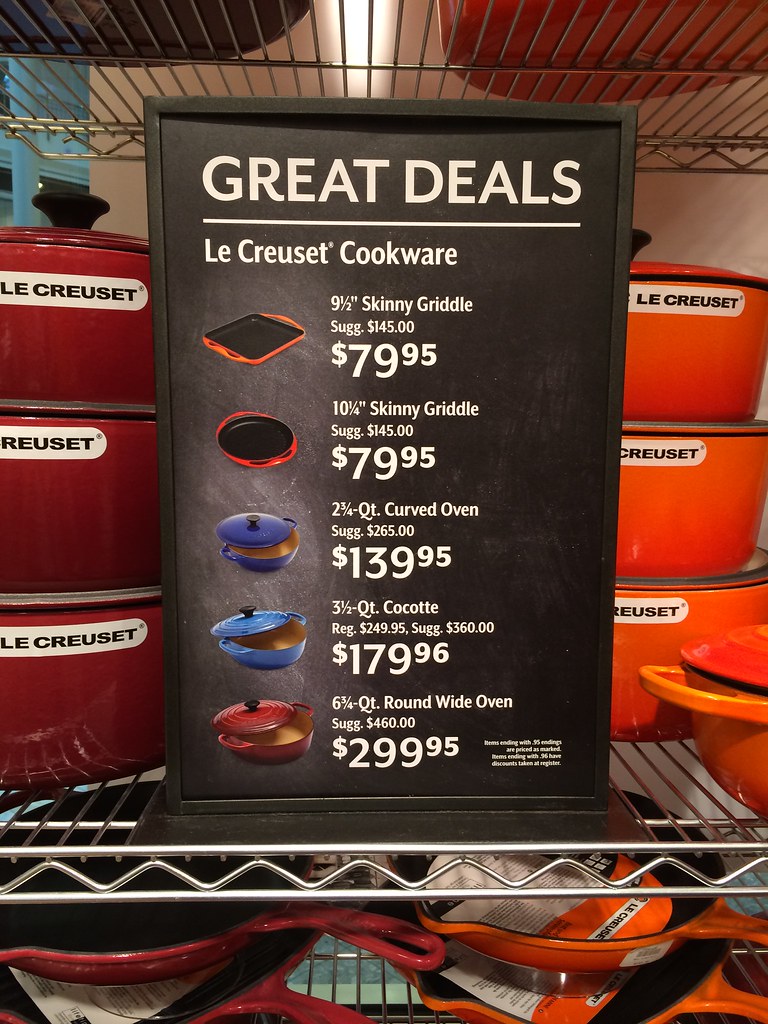This close-up image captures a neatly arranged store display showcasing kitchenware. The display is organized in three tiers, with the bottom rack featuring a variety of pans meticulously aligned. The middle rack, which takes center stage in the composition, primarily displays pots of different sizes and styles. Prominently placed in front of the pots is a rectangular black menu display sign. At the top of the sign, bold white lettering announces "Great Deals." Below this heading, the sign lists five vertical sections, each containing a brief description of a product accompanied by its price, all written in white font for clear visibility. The overall arrangement is thoughtfully structured to highlight the available products and their competitive prices, enticing potential customers with well-organized information.